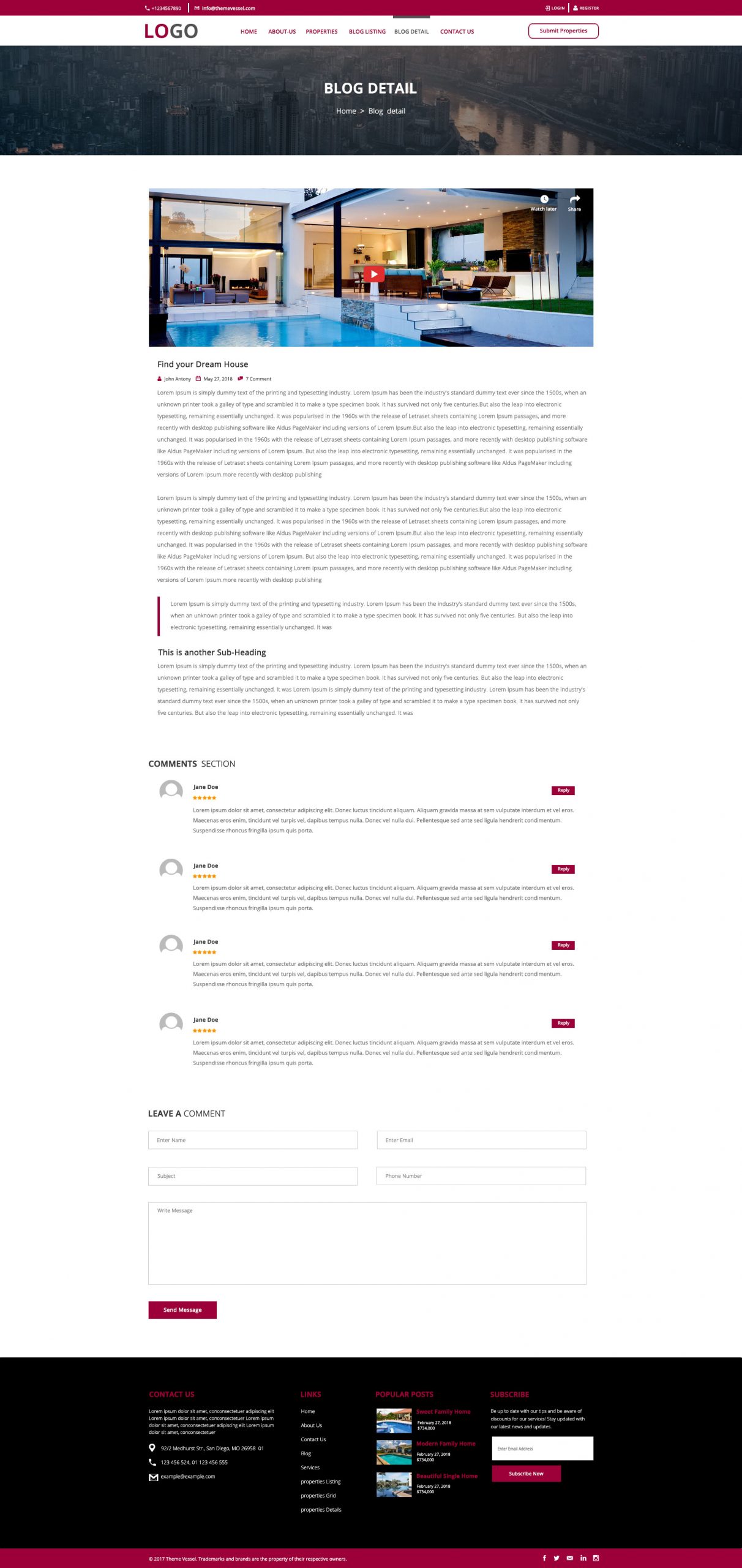The image depicts a distant view of a blog page, making the text somewhat illegible. At the top of the webpage, there is a thin red horizontal line spanning the entire width from left to right. Directly beneath this red line is a slightly thicker white line serving as the menu bar of the website. Towards the left side of this white bar is the word "LOGO" in red font, prominently displayed in a larger size compared to the other text elements. 

Following "LOGO," positioned centrally on the white line, are six menu items, each representing a different section of the website. Toward the right end of this same white bar, a notable larger button is present.

Below the menu bar, there's a thicker gray banner stretching horizontally across the middle of the page, displaying the text "BLOG DETAIL."

In the main content area of the webpage, which is located below the gray banner, there appears to be an embedded YouTube video, indicating that video content is featured as part of the blog post.